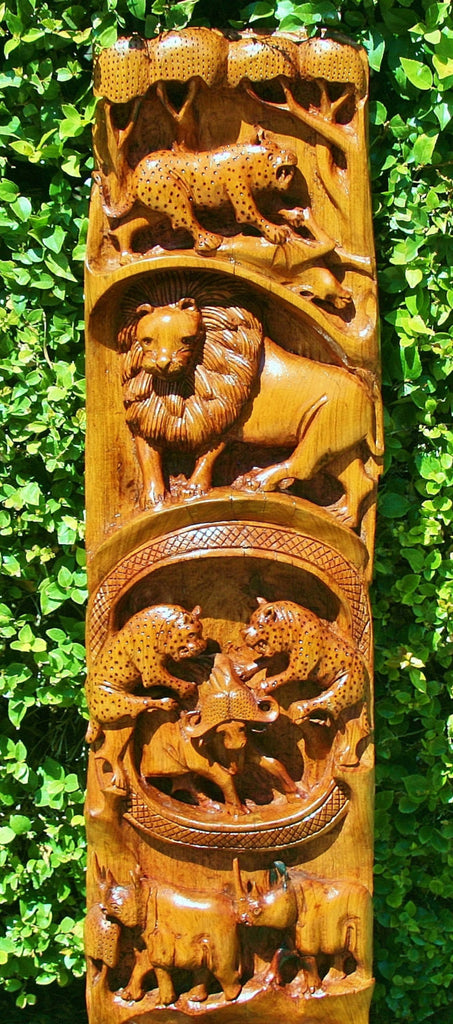This color photo captures a vertical, totem pole-like wood carving set against a background of grass and leafy plants. The carving, crafted from blondish wood with intricate patterning around each animal group, depicts a sequence of wildlife scenes stacked upon each other in a stylized, almost cartoonish manner reminiscent of African art.

Starting from the top, the carving features a leopard under carved trees, facing to the right. Below this, a lion with a large mane is depicted facing to the left, framed within its own section. Lower still, two jaguar-like animals mirror each other on either side of a gnu or water buffalo, capturing a dynamic moment as they appear to be attacking their prey. At the bottom, two rhinoceroses, placed one behind the other, are both carved facing left. Each layer of this elongated, rectangular piece tells a part of a vivid, interconnected wildlife story.